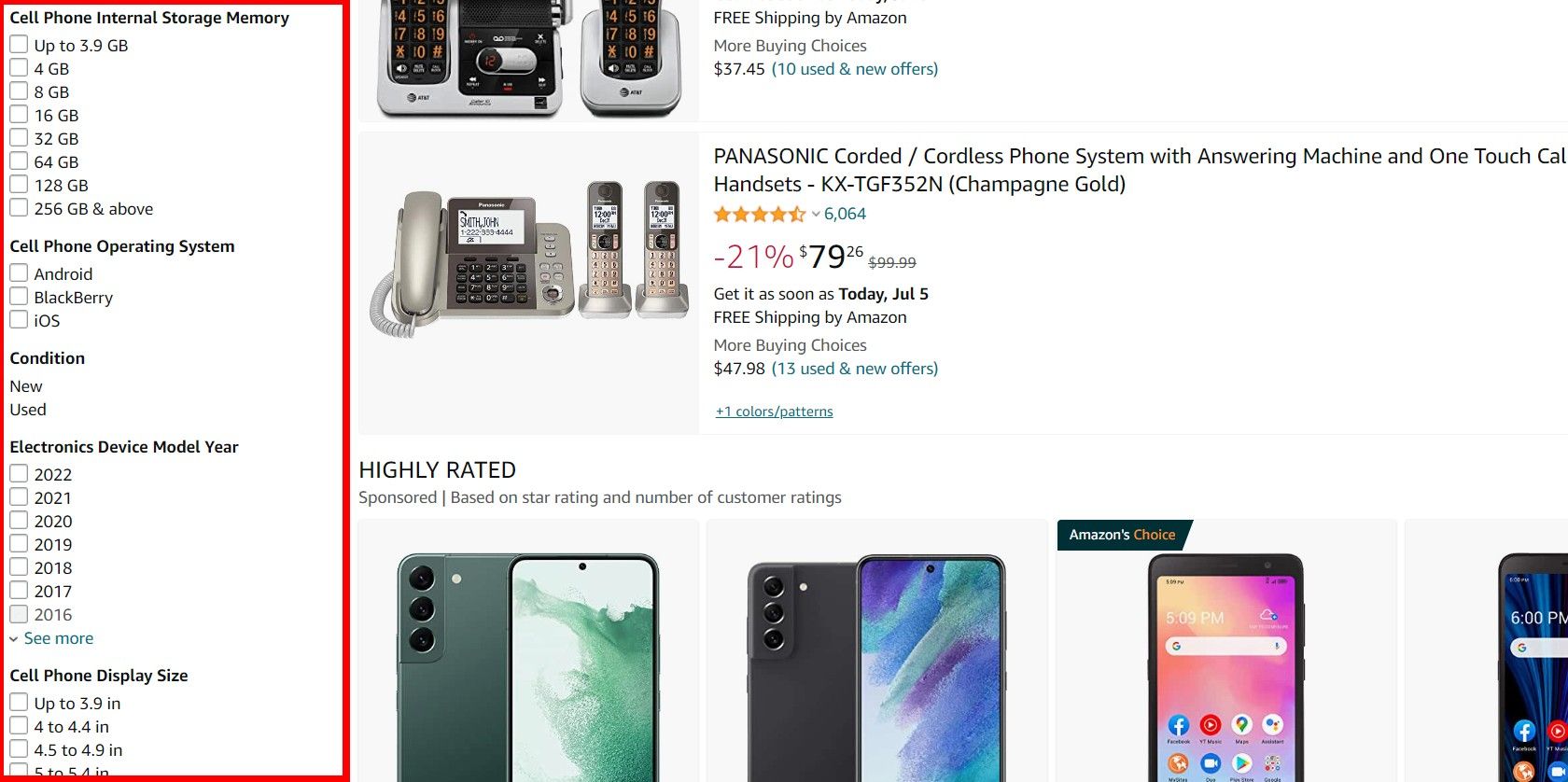A detailed chart on a white background showcases various specifications for cell phones. At the top, multiple categories, each with checkboxes, indicate features like internal storage memory options (3.9 GB, 4 GB, 8 GB, 16 GB, 32 GB, 64 GB, 128 GB, 256 GB and above), none of which are checked. A red rectangle highlights several storage sizes. The chart details various cell phone operating systems, including Android, BlackBerry, and iOS, along with the condition (new) and usage (electronics device). The model years indicated span from 2016 to 2022. A section in blue labeled "More" is visible.

Separately, cell phone display sizes are outlined, ranging from up to 3.9 inches, 4 to 4.4 inches, 4.5 to 4.9 inches, and 5 to 5.4 inches. Accompanying this data is an image of a phone, with text beneath describing it as a "Panasonic corded/cordless phone system with answering machine and one-touch call handsets," model number KXTG.

This well-organized chart offers an exhaustive breakdown of cell phone features and specifications, aiding in easier comparison and selection.